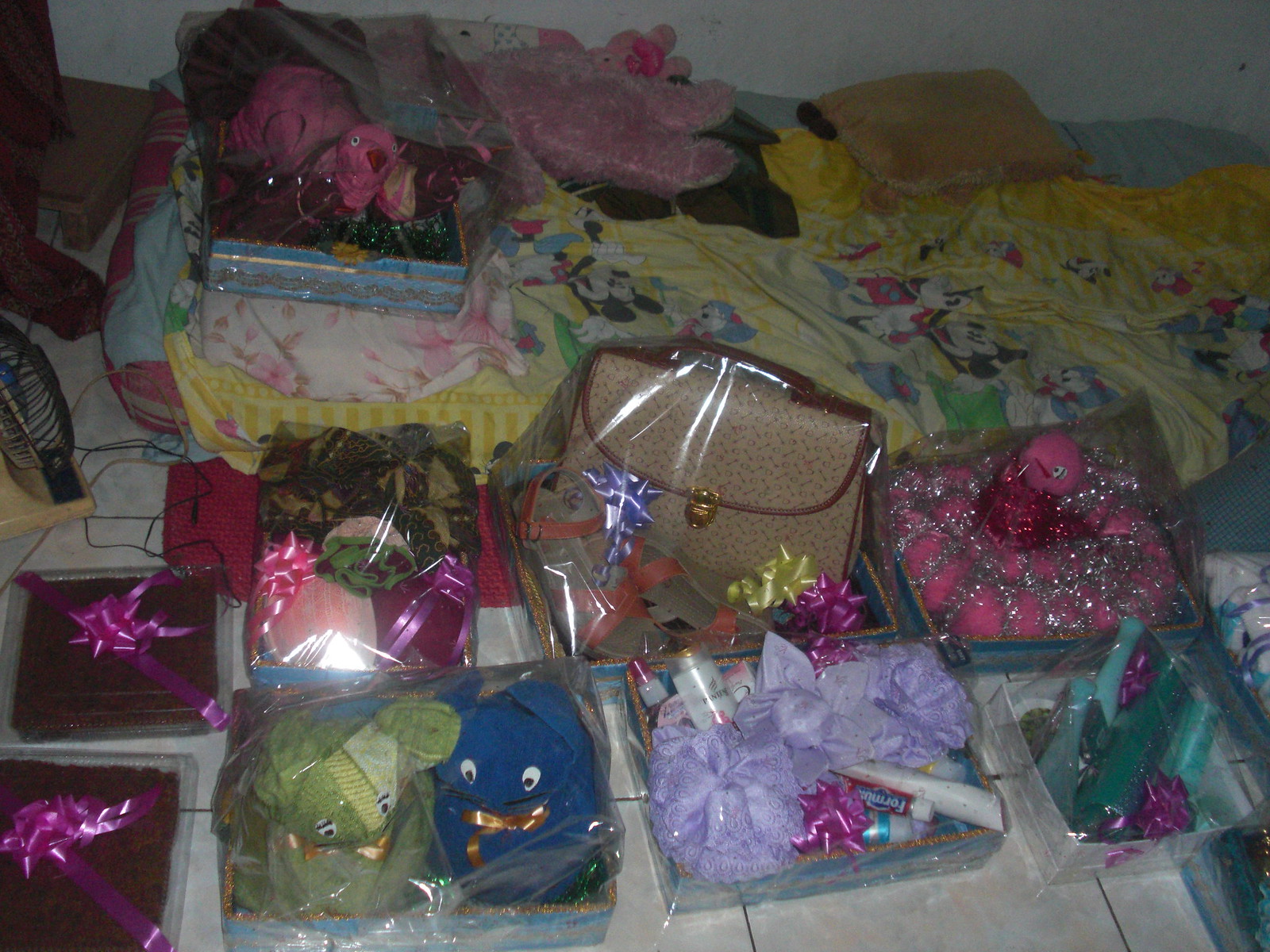In this underexposed, indoor photograph taken in poor lighting, we see a collection of gift baskets and packages arranged on a white-tiled floor. Each rectangular gift basket or box is individually wrapped in clear cellophane and adorned with bows. The scene reveals a variety of contents: a green and blue stuffed animal, a tan and brown purse with brass fittings, and what appears to be cosmetic products including lip balm, nail polish, and possibly four bottles of lotion or perfume. Another tray features pink spheres entangled with tinsel, and yet another contains a large pink stuffed ostrich. Additionally, two small square presents with purple ribbons and bows are visible. In the background, a mattress with a yellow comforter can be partially seen, along with a blanket or throw displaying Mickey Mouse and other characters. Black wires are scattered on the upper left side of the floor, and the overall image lacks any textual elements or clarification, giving it a grainy, dimly lit appearance. This detailed assortment of gift boxes suggests a festivity or event like a raffle or festive giveaway.